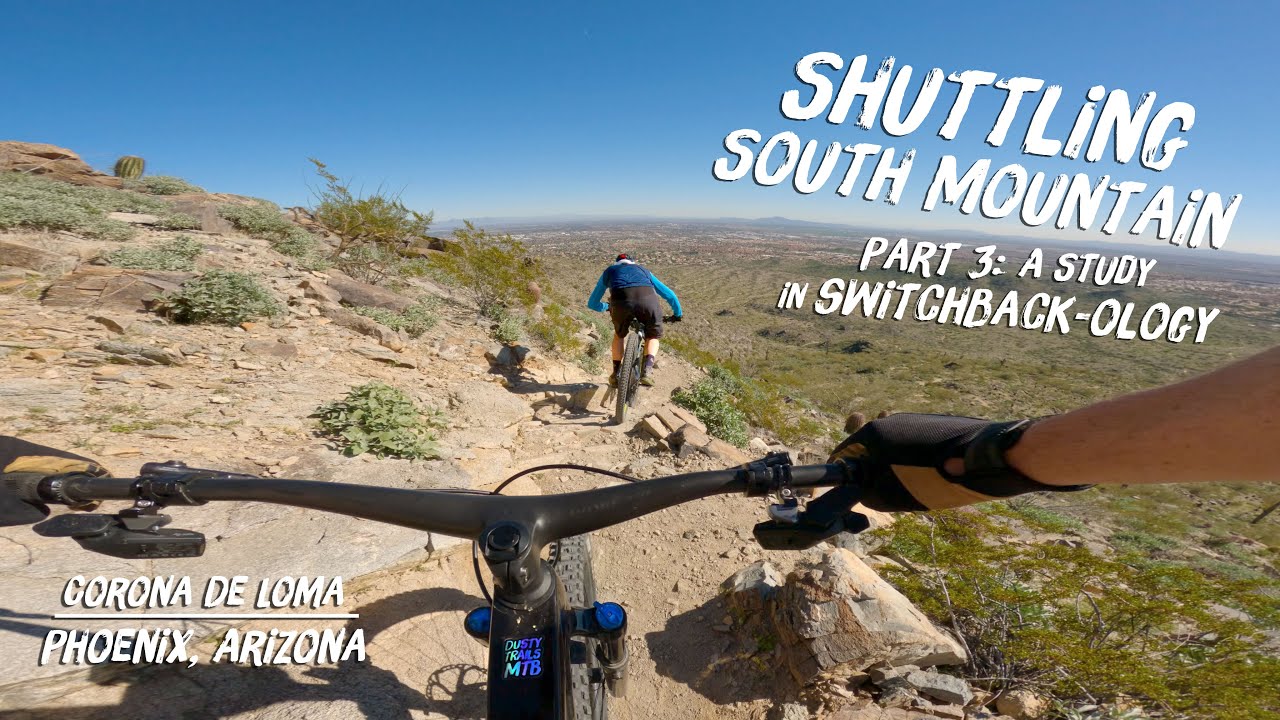The photograph, overlaid with white text, captures a dynamic scene of two mountain bikers navigating a rugged, rocky trail in the Sonoran Desert. The image, which resembles a video thumbnail, prominently features the text "Shuttling South Mountain Part 3, A Study in Switchbackology" in the top right corner, and "Corona de Loma, Phoenix, Arizona" in the bottom left corner. The camera appears to be mounted on the bike of the second rider, providing a detailed view of the handlebars, a gloved hand gripping the right handlebar, and the front wheel. The rider in the foreground, clad in dark shorts and a two-tone blue top, is seen from behind as they ride ahead. The trail, composed of brown sand and rocks, is flanked by desert vegetation such as mesquites and barrel cactus. To the right, a dramatic drop-off reveals a sweeping view of the desert landscape far below, under a vast blue sky. This high-altitude trail appears to traverse the edge of a cliff, adding an element of thrilling adventure to the scene.